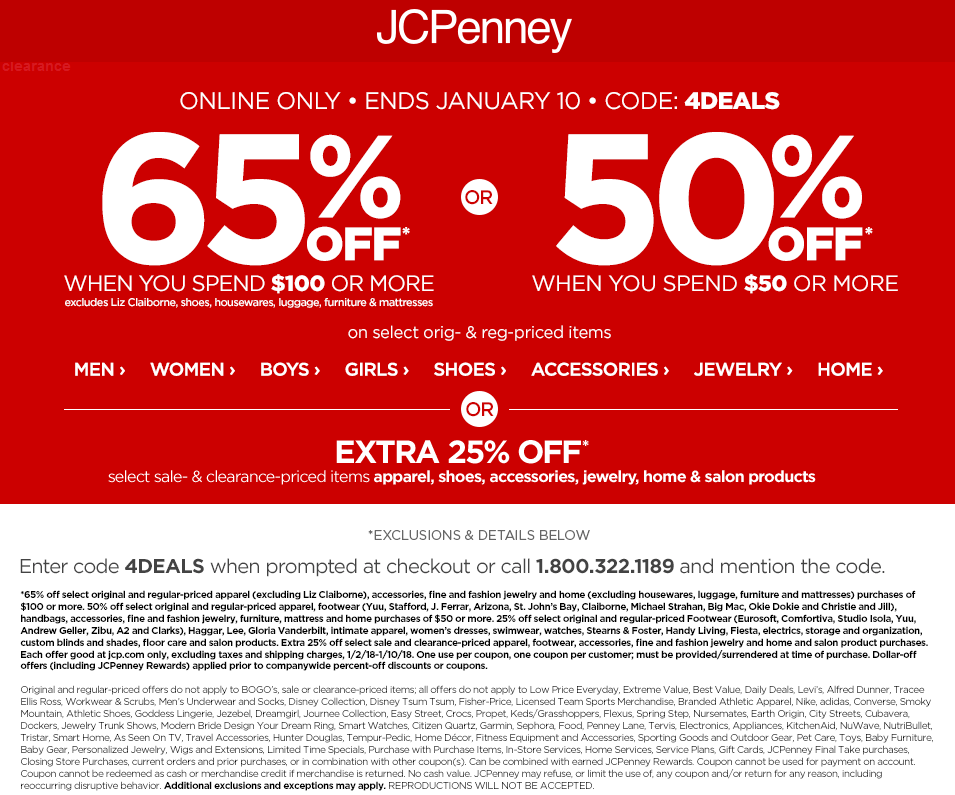This image depicts a detailed JCPenney discount coupon banner, most likely sourced from their website. The coupon, which is the central focus of the image, is rectangular and features a striking red background with all the text in white, ensuring high visibility.

At the very top of the banner, "JCPenney" is prominently displayed, with a note just below that reads "Online Only," followed by "Ends January 10." The discount code "4DEALS" is prominently highlighted beneath this. 

On the left-hand side, the coupon offers a substantial "65% Off" when customers spend $100 or more, with exclusions specified for Liz Claiborne, shoes, housewares, luggage, furniture, and mattresses. There’s also a "50% Off" option for expenditures of $50 or more, applicable to select orange and red-priced items, as mentioned in smaller text underneath.

Further down the banner, a series of small, clickable links guide shoppers to various categories, including Men, Women, Boys, Girls, Shoes, Accessories, Jewelry, and Home. Toward the end, the banner offers an "Extra 25% Off" on selected sale and clearance-priced items across categories such as apparel, shoes, accessories, jewelry, home, and salon products.

Beneath this offer, detailed text against a white background provides specific instructions and additional information: "Exclusions and details below. Enter code '4DEALS' when prompted at checkout or call 1-800-322-1189 and mention the code." Two paragraphs follow, containing further details about exclusions and the workings of the coupon, ensuring customers understand the terms and conditions.